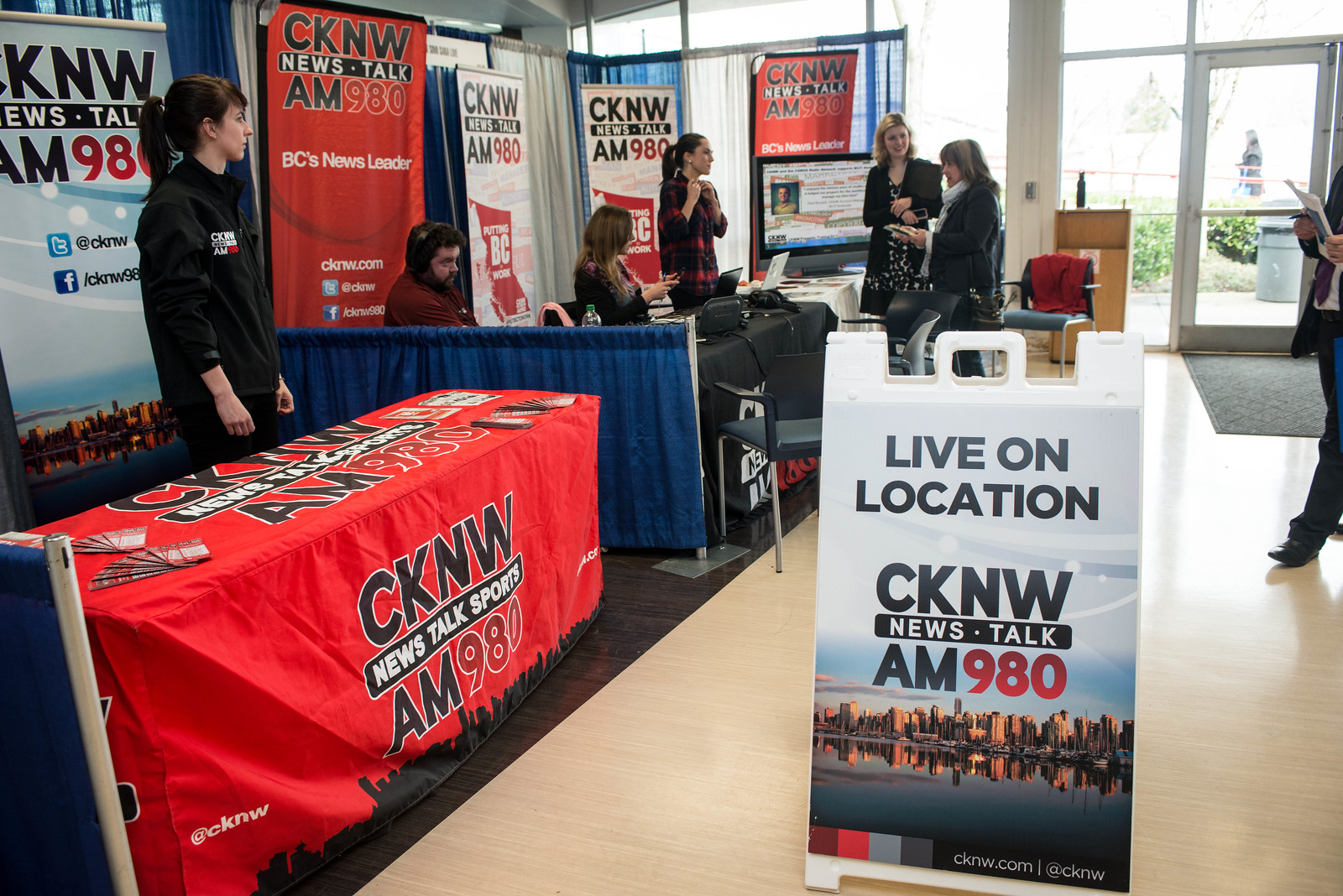The image captures an indoor trade event held in the foyer area at the front of a building. Prominent in the center and illuminated by natural light from nearby glass double doors, are two adjacent booths promoting CKNW News Talk AM 980, BC's News Leader. A banner featuring a city skyline and the text "Live on Location CKNW News Talk AM 980" is prominently displayed at the center of the photo. In the left booth, a woman dressed in black is engaging attendees, with brochures spread out on her table covered in a branded tablecloth. Beside her booth, to the right, three women equipped with laptops are conversing with interested visitors. A man wearing headphones, presumably participating in a live radio broadcast, is also visible in the background. The event space, detailed with blue barriers and additional promotional posters, exudes a bustling atmosphere as CKNW News Talk AM 980 stations demonstrate their offerings and interact with potential listeners.